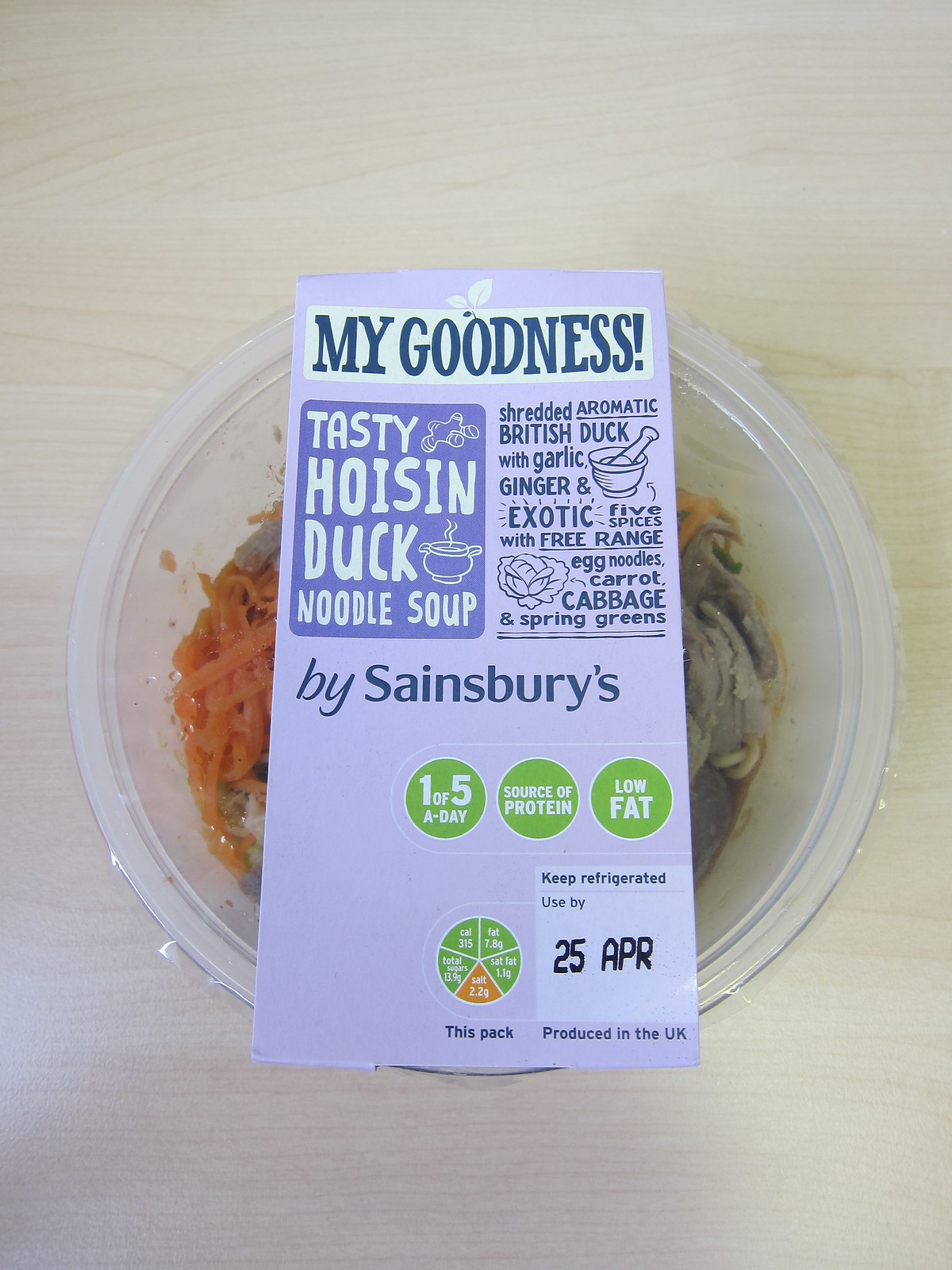This image showcases a packaged meal from Sainsbury's: Tasty Hoisin Duck Noodle Soup. The meal is presented in a clear plastic bowl sealed with plastic wrap and adorned with a light blue cardboard label that wraps around the bowl. The label prominently features the phrase "My goodness!" in darker blue letters, along with the product name. Inside the bowl, you can faintly see some of the ingredients, including shredded aromatic British duck meat tinted brown, orange carrots, and bits of other components. The detailed label describes the meal as consisting of shredded aromatic British duck with garlic, ginger, and exotic five spices, paired with free-range egg noodles, carrots, cabbage, and spring greens. It indicates that the meal is a source of protein, low in fat, and counts as one of the recommended five-a-day servings of vegetables. The packaging advises to keep the meal refrigerated and to consume it by the 25th of April. Nutritional information, including salt, calories, total sugars, fat, and saturated fat content, is also provided. This product is produced in the UK.